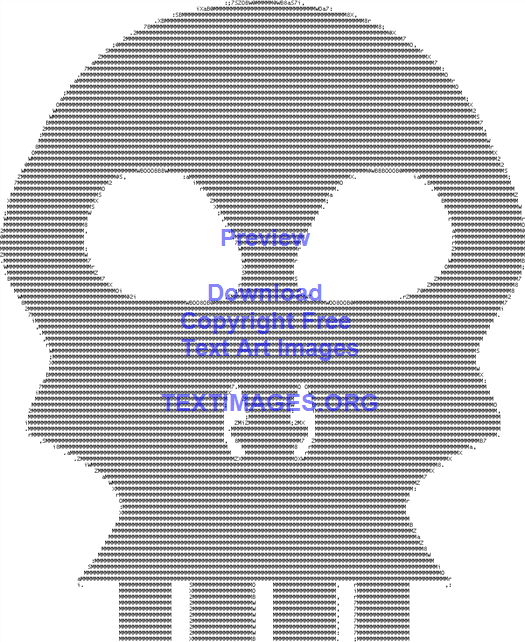This ASCII art image showcases a large, perfectly symmetrical skull with distinctive features, including high-positioned eye sockets, unique nostril shapes, and angular, square-looking teeth at the bottom. The entire skull forms a circular shape and is meticulously shaded using black text characters. On top of the skull, a purple watermark provides information, reading "Preview Download Copyright Free Text Art Images at textimages.org," with "TEXTIMAGES.ORG" prominently in all capital letters. This detailed text art is available for free download from the mentioned site, embodying a mix of traditional skull imagery and an alien twist.